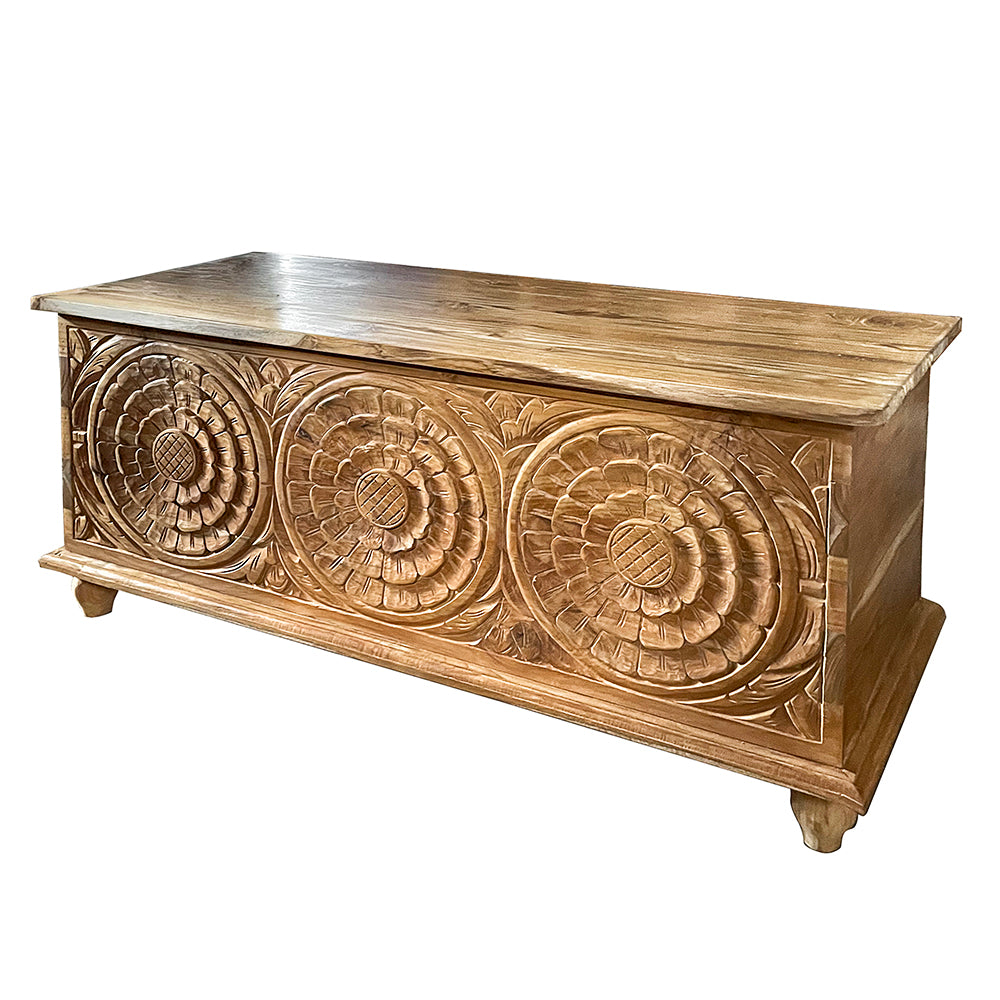This is a color photograph of a wooden chest or credenza set against a plain white background, showcasing a piece that might also be interpreted as a coffee table or a vintage-style cabinet. The wood is intricately hand-carved with a detailed, 3D design that features three large, round stylized flowers, each with a central knob. The wood grain showcases a range of shades from light brown to medium brown to dark brown, with subtle white streaks, giving it a rich and dynamic appearance. The top of the chest is plain wood, while the base protrudes slightly and the front legs are short and visible, adding to its sturdy presence. The entire piece is well-polished, exuding an antique feel, and demonstrates the craftsmanship and care taken in its creation, making it a striking and potentially valuable item.